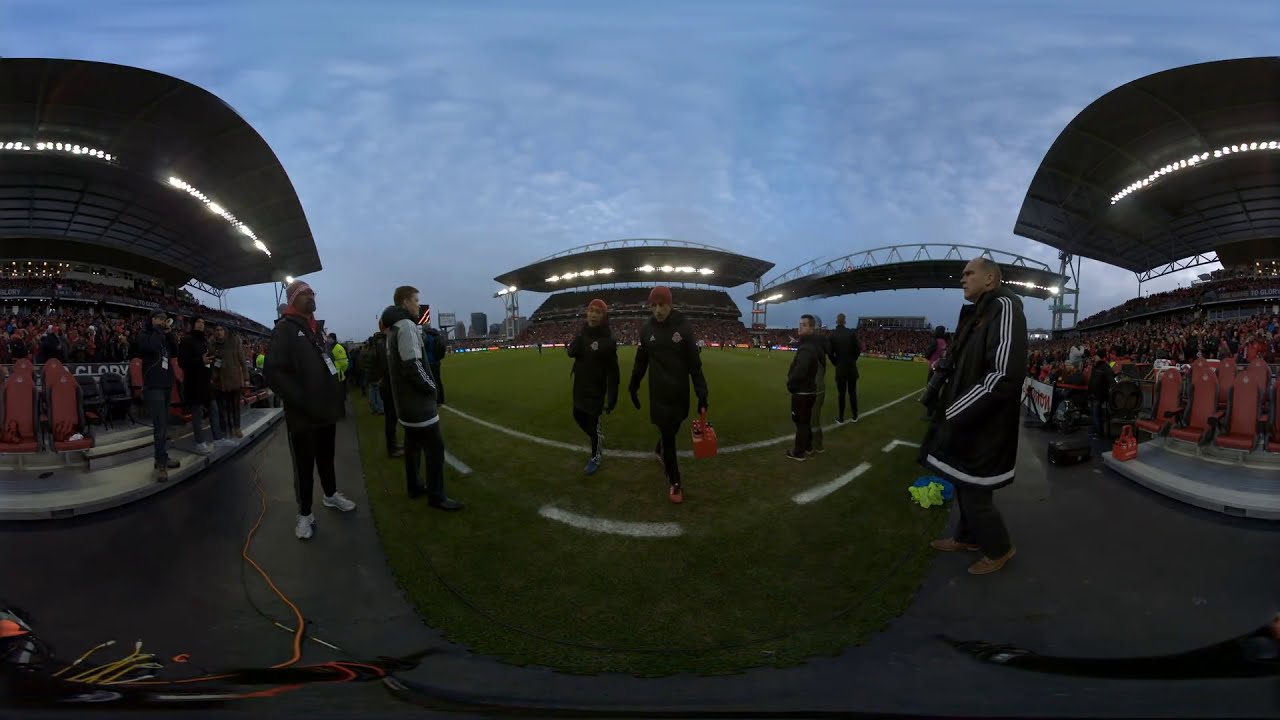The image captures an outdoor sports stadium in the later evening or possibly early morning, under a dark, overcast sky punctuated by high clouds. The stadium's green turf field features a white solid painted line and curved white dotted stripes. Stadium lights are illuminated, casting an ethereal glow over the scene. The stands, segmented into four distinct sections with red seats, have a bubble-like effect due to the photo's filter, creating a curved, almost panoramic view.

The field is populated with numerous individuals, likely players and spectators, dressed predominantly in black long-sleeve tops and pants, some wearing hats and dark coats with logos. One individual is seen carrying a red box, while many others stand with their hands in their pockets, suggesting a cold day. The ambient lighting from the stadium lights, combined with the twilight or early morning conditions, gives the entire scene a moody yet vibrant atmosphere.